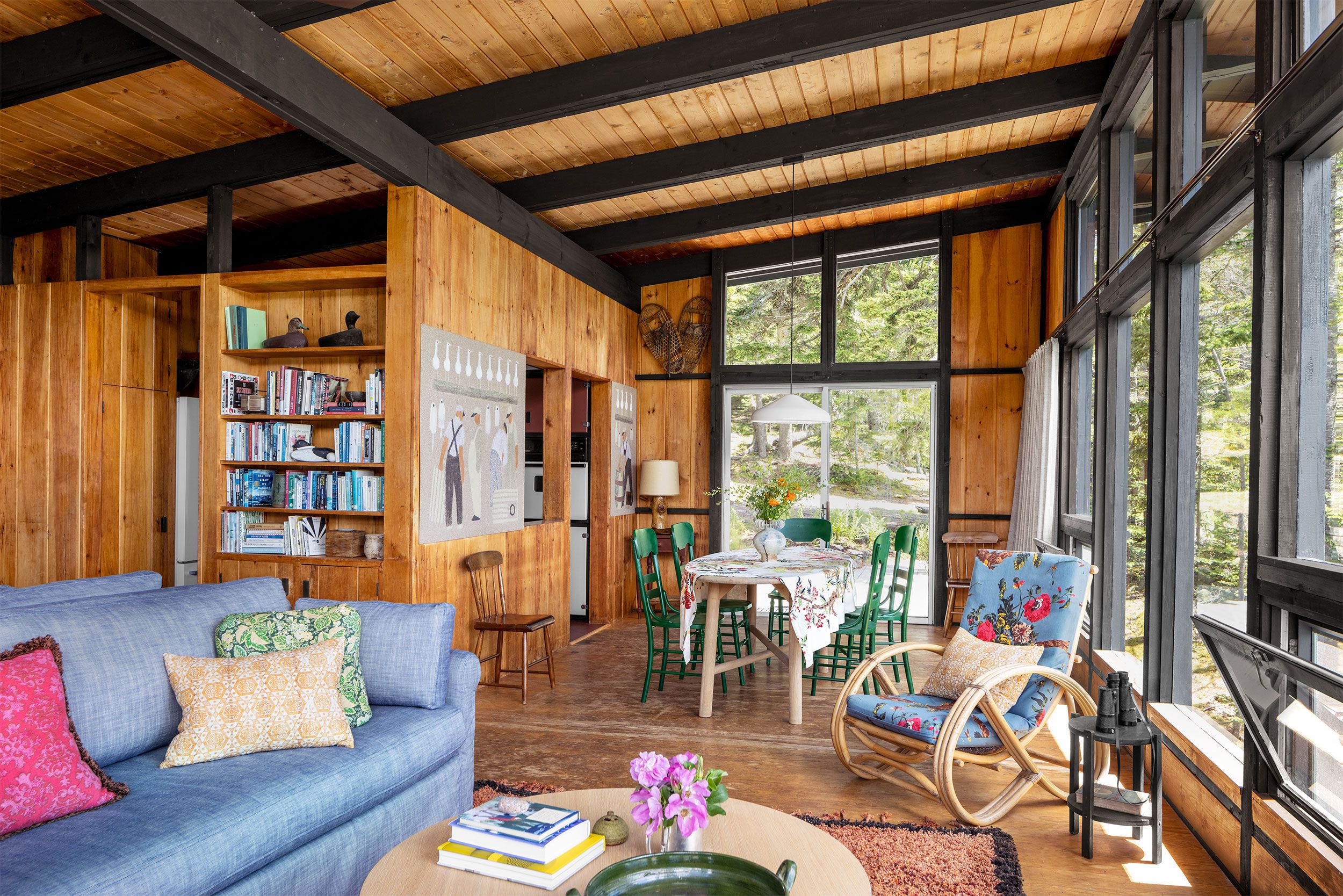The sunlit interior of the room features a harmonious blend of rustic charm and cozy furnishings. The walls and ceiling of this sunroom are crafted from vertical and perpendicular planks of rich, chestnut-colored wood, adding a warm and inviting feel. A series of large windows with black inner spacing dividers flood the space with natural light, enhancing the room's earthy tones. Prominently positioned on the bottom left is a bright blue sofa adorned with colorful patterned pillows in red, yellow, and green. In front of the sofa sits a small, circular coffee table made of light wood, elegantly decorated with a vase of purple flowers, a stack of books, and a bowl. To the right, a blue rocking chair with floral patterns complements the cozy seating arrangement. Adjacent to this chair is a slightly open door revealing a glimpse of a refrigerator, suggesting a connection to the kitchen area. A bookshelf filled with books further enhances the sunroom's ambiance, while two paintings add a touch of artistic flair on the wall beyond the corner. In the back, you can see a sliding screen door inviting you to explore further, while the scattered green and black accents provide a modern contrast to the naturally finished wood, making this sunroom a perfectly balanced retreat.